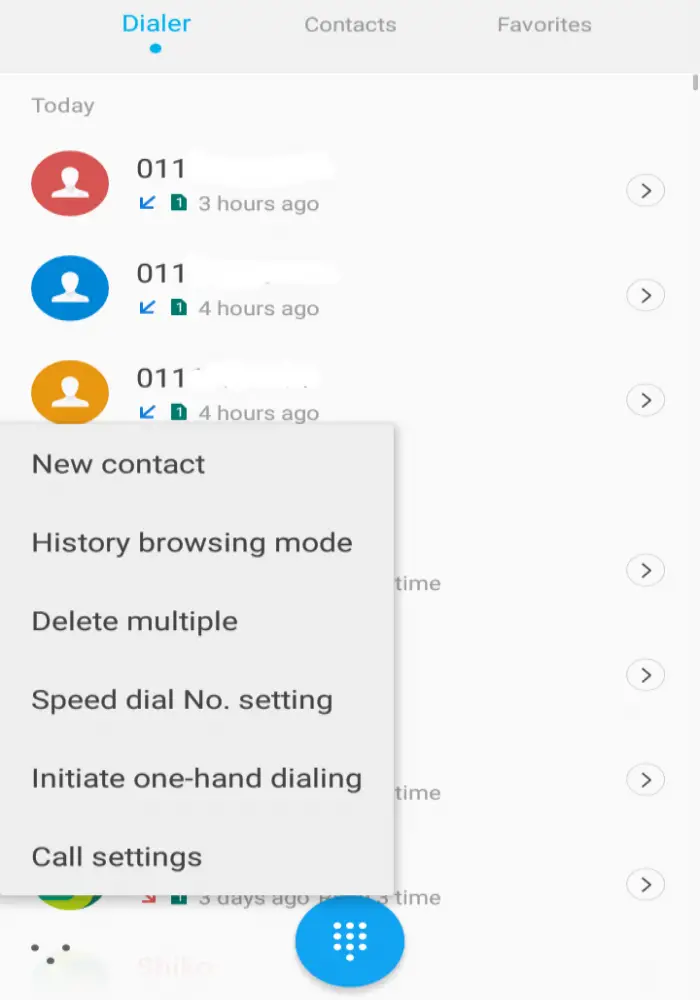The image depicts the interface of a phone dialer application. At the top, there are three tabs labeled 'Dialer,' 'Contacts,' and 'Favorites.' The 'Dialer' tab is highlighted in blue, while the other two are gray, all set against a light gray background strip. Below this strip, the background lightens further.

On the upper left corner of the main section, it says 'Today.' Below this, there are several entries representing recent calls. Each entry includes a circular icon with different colors and icons:

1. A red circle with a white person icon, accompanied by '011,' a blue arrow pointing downward to the left, the number '1,' indicating a call from three hours ago.
2. Another entry with a blue person icon, featuring the same '011' and blue downward-left arrow, denoting a call from four hours ago.
3. A yellow circle with a person icon, also marked with '011' and the downward-left arrow, indicating another call from four hours ago.

Overlaying these entries is a pop-up menu with options, including 'New Contact,' 'History Browsing Mode,' 'Delete Multiple,' 'Speed Dial Number Setting,' 'Initiate One-Hand Dialing,' and 'Call Settings.'

At the bottom center of the screen is a blue circle containing ten dots arranged in a square formation with an additional dot below it. On the bottom left, there are three black dots forming an inverted V shape, pointing downward.